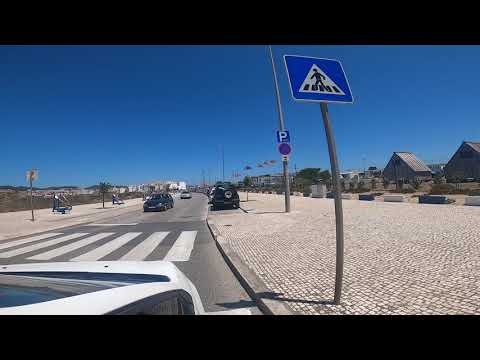This is a photograph of a bustling city street under a clear, sunny blue sky with no clouds, suggesting a bright, perhaps summer day. The image captures the front part of a white car approaching a crosswalk in the middle of the road. Dominating the right side of the image is a sandy-colored, tile-paved walkway lined with various street signs. The foremost sign is a blue square with a white triangle and a black icon of a man walking on a crosswalk, indicating pedestrian crossing. Just behind it stands another pole with a blue parking sign marked by a large white "P".

In the distance, a couple of darker-colored cars appear to be driving towards the viewer, reinforcing the sense of a two-lane road. On the distant right side, there are A-frame and barn-shaped buildings, set about 100 yards from the road, with greenery and trees around them. The road itself is lined and shows traffic moving in both directions, indicating a moderately populated area. The left side of the photo includes a grey road and a distant walkway highlighted by greenery and a visible horizon. Overall, the image presents a slice of busy, yet picturesque urban life.